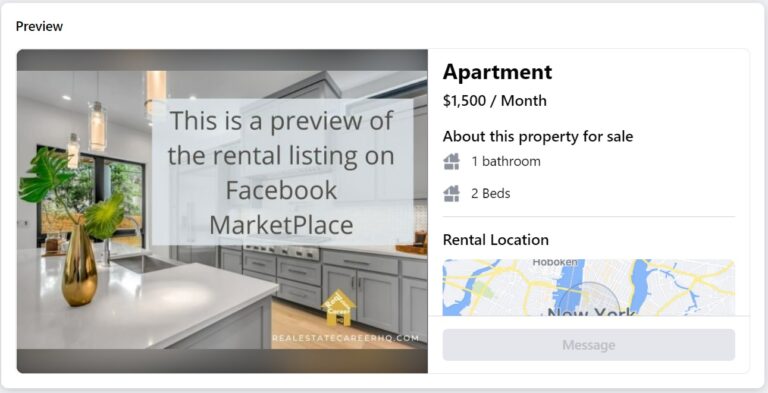**Detailed Caption:**

This image is a detailed screenshot of an apartment listing available for rent, prominently displayed against a white background. The focal point on the left side is a large photograph that showcases the kitchen area of the apartment. The kitchen features modern gray cabinets, complemented by sleek white countertops and a light wood floor. Central to the kitchen is an island equipped with a sink, adorned with a stylish gold vase filled with green leaves. Above the island are three elegant drop lights, accompanied by recessed can lights to enhance the illumination. In addition, there are sliding glass doors that likely lead to an outdoor space, adding a touch of openness and natural light to the area.

To the left of the sink, there is a gas stove with additional cabinetry and drawers below, providing ample storage and functionality. The image has textual elements, including the word "Preview" in black at the top left corner, indicating that this is a preliminary view of the listing. A gray box superimposed on the image states, "This is a preview of the rental listing on Facebook Marketplace."

The listing details reveal that this is a two-bedroom, one-bathroom apartment available for $1,500 per month. There is also an included map highlighting the rental location in New York, ensuring prospective tenants can easily identify the geographic area. Additionally, the image features a yellow house icon with the website "realestatecareerhq.com," suggesting a connection to online real estate resources.